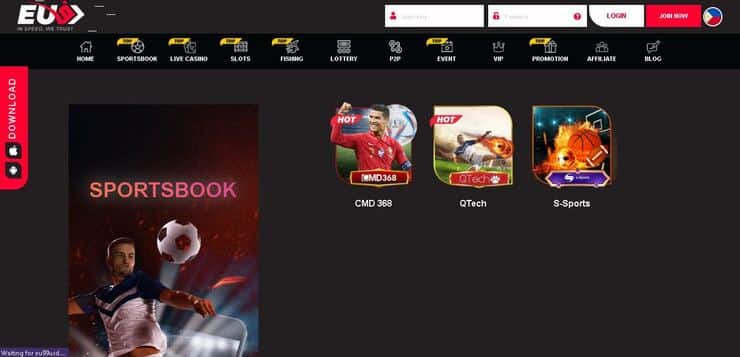Screenshot of the EUG Sports Book and Gambling Website:

The image is a screenshot from the EUG sports book and gambling website, which combines slots and sports betting options. In the top left corner, the website's logo "EUG" is prominently displayed, with the letters "EU" in white and the letter "G" in red, tilted slightly to the right. Below the logo, a black header bar spans the width of the page, featuring icons for Home, Sports Book, Live Casino, Slots, Fishing, Lottery, P2P, Event, VIP, Promotions, Affiliate, and Blog.

Above this header is a horizontal strip containing user interface elements: two white input boxes for "Username" and "Password," alongside a Login button and a red "Join Now" button located at the top right corner. Additionally, the flag of the Philippines is displayed in a small circular icon.

The website's background is dark gray, creating a stark contrast with the other elements. On the right side of the screen, a vertical banner advertises the Sports Book, featuring a computer-generated image of a soccer player kicking a ball. Another vertical red stripe on the far left side reads "Download."

In the main body of the webpage, three icons are prominently featured:
1. **CMD368** – represented by an image of a soccer player.
2. **QTEK** – showcasing a soccer player kicking a flaming soccer ball.
3. **sSports** – depicting a soccer ball and a basketball with a flame behind them set against a dimmed basketball court.

The arrangement and vivid imagery clearly emphasize the website's focus on sports and gambling activities.